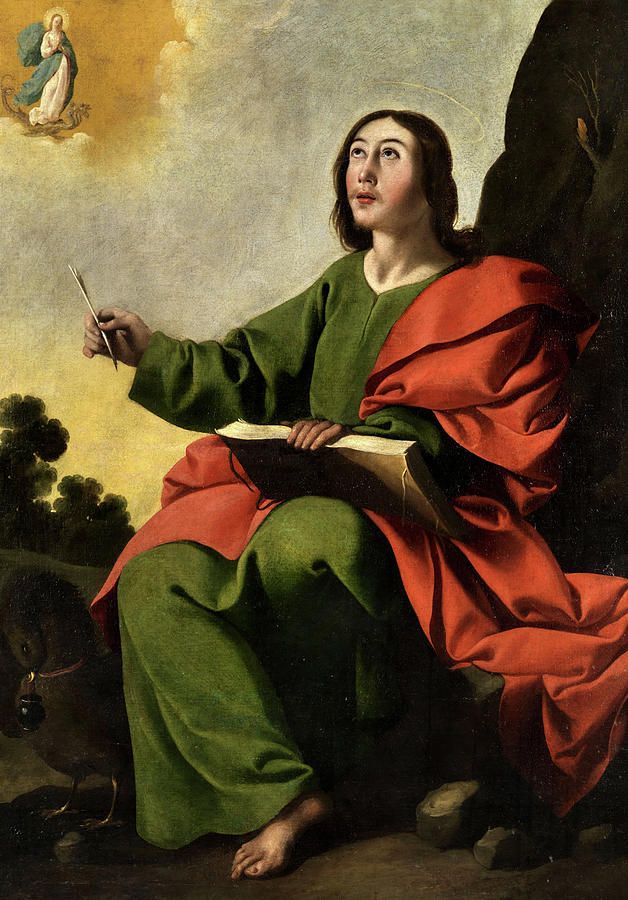The painting depicts a holy man, likely a monk or saint, sitting barefoot on a rock. He has long dark brown hair and is adorned in an olive-green robe. A voluminous red cloth drapes over his right shoulder and flows down to his feet. The man is intently looking upward toward the upper left corner of the painting. In his left hand, he holds an open book, gripping it at the middle, while his right hand holds a quill-like pen. The background features a serene sky with a glowing angel descending on a cloud, wearing a white and blue robe, and radiating divine light. Additionally, a faint halo encircles the man's head, emphasizing his holy nature. A small, brown animal, possibly a chicken, stands next to him, adding a touch of life to the scene.